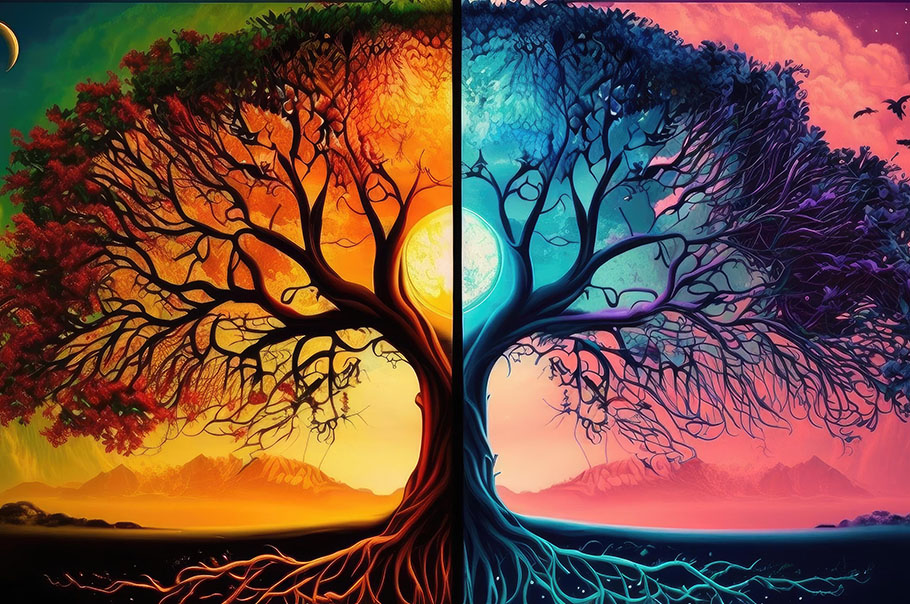This image is a detailed and vibrant depiction of a large tree, symmetrically split down the middle to showcase two contrasting color schemes, possibly representing different seasons or symbolic meanings. The left side of the image features a tree with warm orange tones in its branches and leaves, set against a backdrop where the sky transitions from greenish-blue at the top to yellowish-orange at the bottom. The background also includes dark orange-yellow mountains. On this side, the ground beneath the tree reveals visible orange roots, suggesting they are above ground.

In sharp contrast, the right side of the image showcases cooler blue and purple hues in the tree's foliage and root system. The sky on this side exhibits pinkish-purple shades, both at the top and bottom, with the mountains reflecting these colors. Centrally, the image features a glowing celestial body—likely a moon or planet—that is split along the vertical divide; appearing golden yellow on the left and a bluish-white on the right.

The tree itself closely resembles an oak with plenty of visible branches and leaves. The dual-toned roots are explicitly shown, further enhancing the symmetry and artistic impact. Underneath and around the tree, the contrasting color palettes create a vivid display that may symbolize opposing forces or the cyclical nature of life.